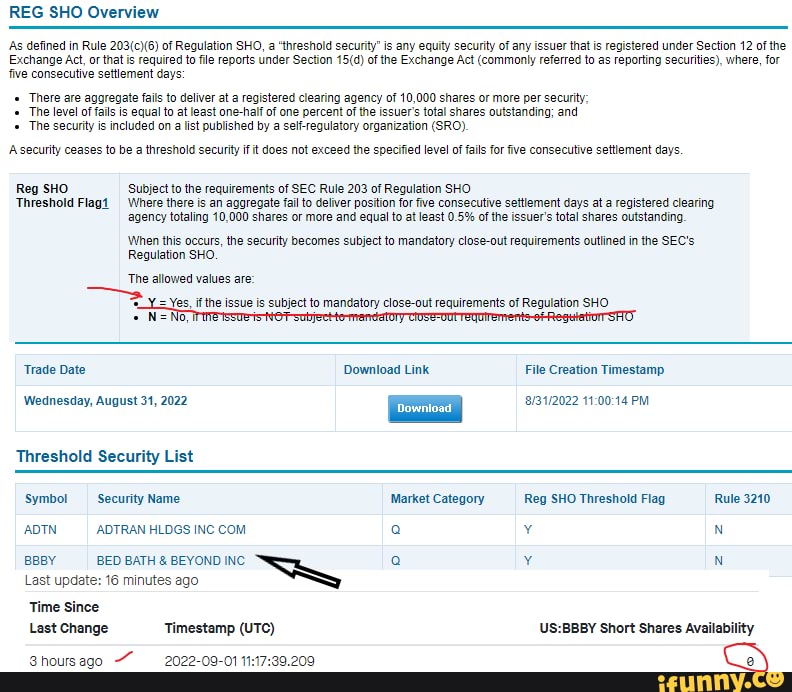**Caption:**

In the upper left corner, the image features the blue text "REG SHO Overview." Just below this title is an informational paragraph spanning two to three lines, followed by three black bullet points.

Underneath the bullet points, a statement reads: "A security ceases to be a threshold security if it does not exceed the specified level of fails for five consecutive settlement days." Below this text, a large blue square is prominently displayed. To the left of the square, in capitalized text, it says "REG SHO." This text is underlined and accompanied by a red arrow.

The explanation continues: "Y = Yes if the issue is subject to mandatory closeout requirements of Regulation SHO," which is underlined. Below this, a line has been struck through another section that reads: "N = No if the issue is not subject to mandatory closeout requirements of Regulation SHO," marked in red.

Further down, the image provides a trade date of "Wednesday, August 31st, 2022," followed by a "Download link" with the word "Download" inside a square box. Proceeding this is the category "Threshold Security List," with a black arrow pointing towards "Bed Bath & Beyond Incorporated." In the lower right corner, the number zero is circled in red.